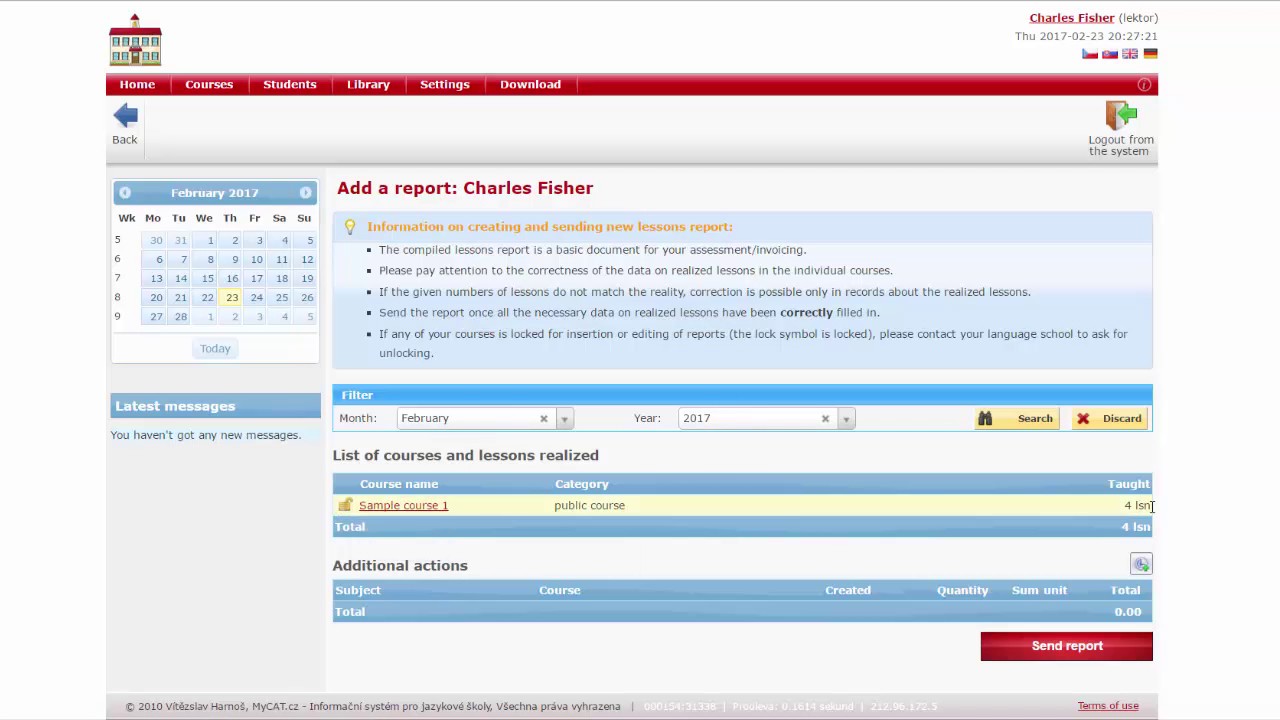A detailed screenshot of a desktop computer showcasing a website interface. At the top of the screenshot, there is an illustration of a house with a red roof on the left side. To the right of the house graphic, the name "Charles Fischer" is prominently displayed in red ink, along with the date "Thursday, 2017 February 2023" and the time "20:27:21". Nearby, there are flags representing different countries or options.

Beneath this, a red navigation bar features several options in white ink, including "Home," "Courses," "Students," "Library," "Settings," and "Downloads." On the left side, there's a green arrow pointing left that says "Back." Another green arrow points towards what appears to be a book or door, labeled "Log Out from the System."

Further down, an open calendar is visible, specifically set to February 2017. The calendar has a white background with black ink for the dates, and some numbers are highlighted in blue. The current date is indicated with "Today" marked. 

Under the calendar are sections showing "Latest Messages," with the note "You haven't gotten any new messages." It also includes options to "Add a Report," "Filter," and "Additional Actions," all referenced near "Charles Fischer" in red ink again.

At the bottom, there's a red button labeled "Send Reports" in white ink. The overall design is clean and structured, providing quick access to various functionalities and information.